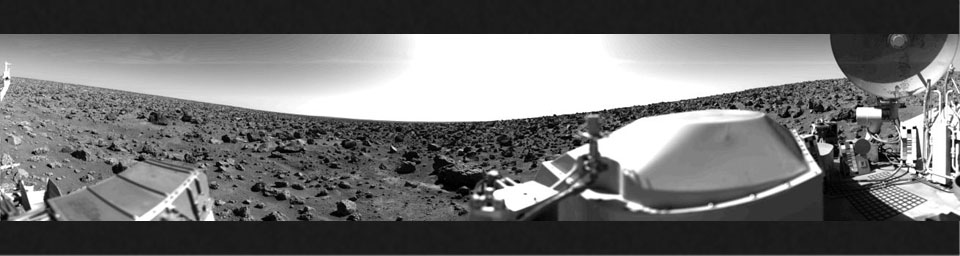This black and white photograph captures a panoramic view of a rocky desert surface, detailed with various elements. In the foreground, a large hatch is prominently visible, lying amidst the rough terrain. To the right, metal equipment is stationed, interconnected by extending hoses, hinting at its technical and possibly space-related purpose. Additional equipment is scattered off to the left, including an object resembling a tank and some other machinery. The center field of rocks stands out as particularly dark, situated under a large glare likely emanating from the sun. Hovering above this glare is a cloudy sky, adding to the stark contrast of the scene. Black horizontal bands frame the image at the top and bottom, adding a sense of encapsulation. In the upper right-hand corner, a pair of circles—one dark gray and one light gray with a black center—are subtly noticeable, possibly part of the equipment or providing some perspective. The overall composition of dirt, rocks, and metal constructs evokes an otherworldly atmosphere, intensifying the desolate and technologically advanced feel of the landscape.